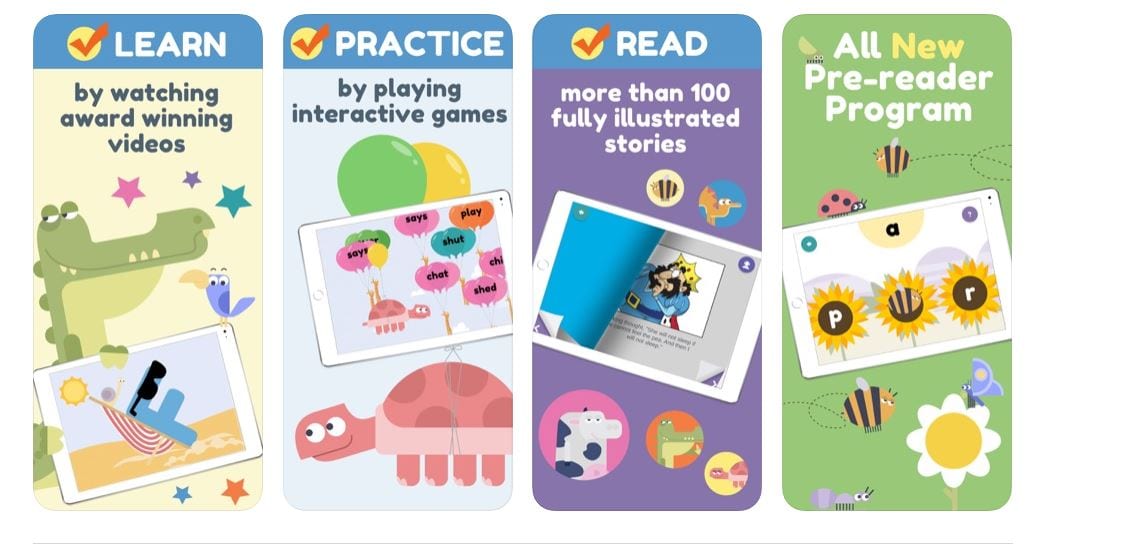This is a horizontal advertisement image for an educational gaming system designed to be accessed online via computer or smart device. The advertisement is divided into four vertical, rounded rectangles, each featuring a distinct aspect of the learning experience.

1. The first rectangle has a blue top section with the word "LEARN" in white letters. Below it, a yellow circle with a reddish-orange checkmark is present. The main section is beige and states, "by watching award-winning videos" in blue text. The visual includes an illustration of an alligator holding a picture of a sailboat, accompanied by stars and a bird.

2. The second rectangle mirrors the top design of the first, but with the word "PRACTICE" in white letters. The background here is light blue and reads, "by playing interactive games." It features an illustration of a turtle with balloons, each balloon containing a word.

3. The third rectangle continues with the same top design, but with the word "READ." The background is purple and mentions "more than 100 fully illustrated stories" in white letters. The visual representation here includes a book surrounded by various animals within circles.

4. The final rectangle has a green background with the text "ALL NEW PRE-READER PROGRAM." The illustration includes ladybugs, flowers, and bees, suggesting different games focused on word learning. 

Each section highlights a unique component of the learning system, emphasizing its comprehensive and interactive approach to education.